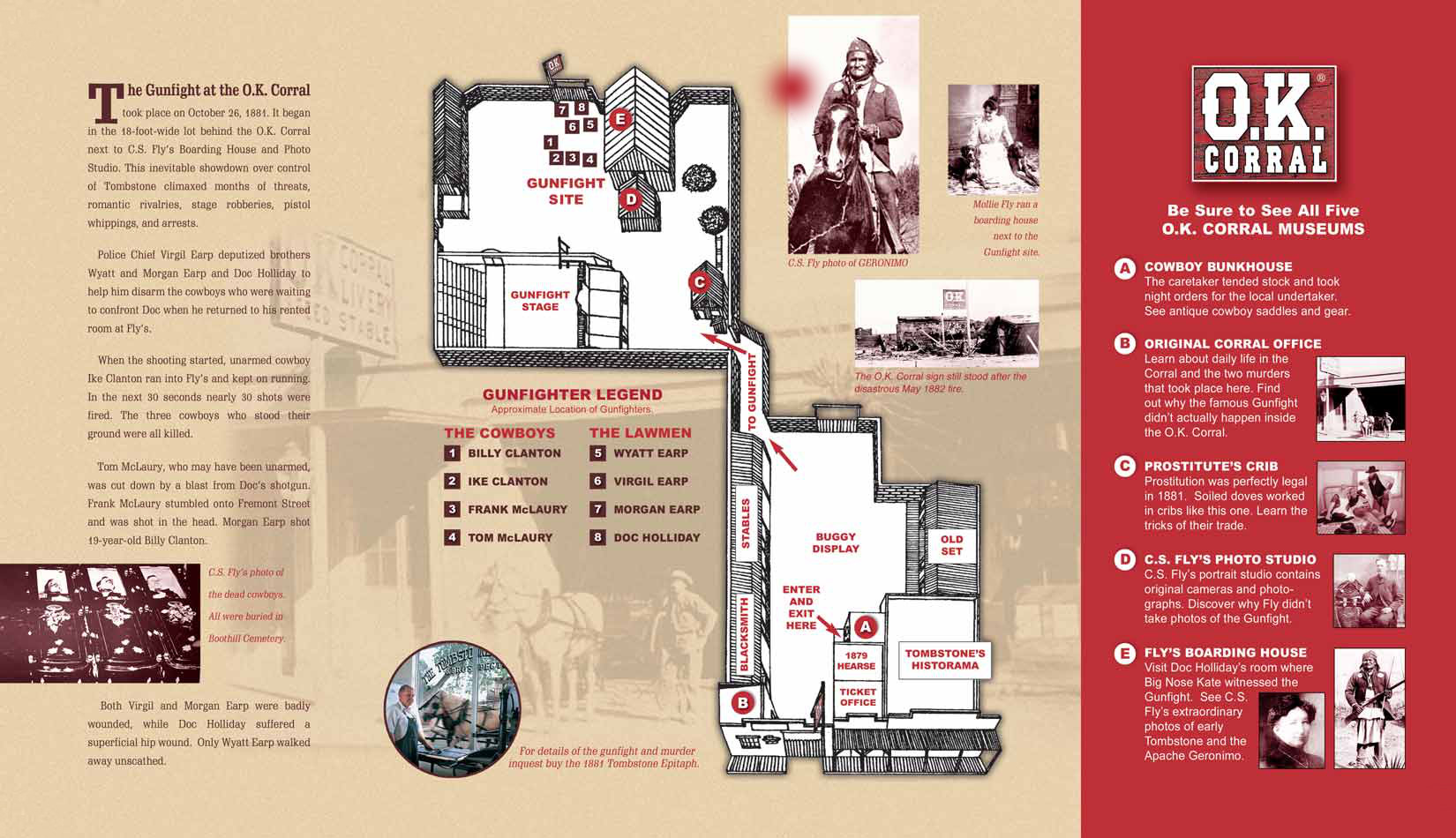The image presents an informational display or pamphlet about the Gunfight at the O.K. Corral, likely seen at the O.K. Corral Museum. The left two-thirds of the display set against a light tan background includes detailed text describing the shootout that occurred on October 26, 1881. It features C.S. Fly's historic photo of the dead cowboys, who were buried in Boot Hill Cemetery, situated at the bottom left. In the center, there's a comprehensive diagram titled "Gunfighter Legend," marked in red font, showing the gunfight stage and exact locations of key players like Wyatt Earp, Virgil Earp, Morgan Earp, and Doc Holliday.

Amidst these details is a circular image with the caption, "For Details of the Gunfight and Murder Inquest by the 1881 Tombstone Epitaph," featuring a man with a horse. The top right features an image of a Native American on a horse, labeled "C.S. Fly's Photo of Geronimo," and adjacent to it, a photograph of Molly Fly in a white dress with a dog, marking her residence next to the gunfight site. Below, a rectangular black and white photo shows the O.K. Corral sign post-May 1882 fire. The left side contains additional text and another continuation of the "Gunfighter Legend" diagram.

The right third of the image has a red background and emphasizes visiting all five O.K. Corral museums: Cowboy Bunkhouse, Original Corral Office, Prostitutes’ Crib, C.S. Fly's Photo Studio, and Fly's Boarding House, each followed by descriptive paragraphs and corresponding photographs of the people and places referenced.